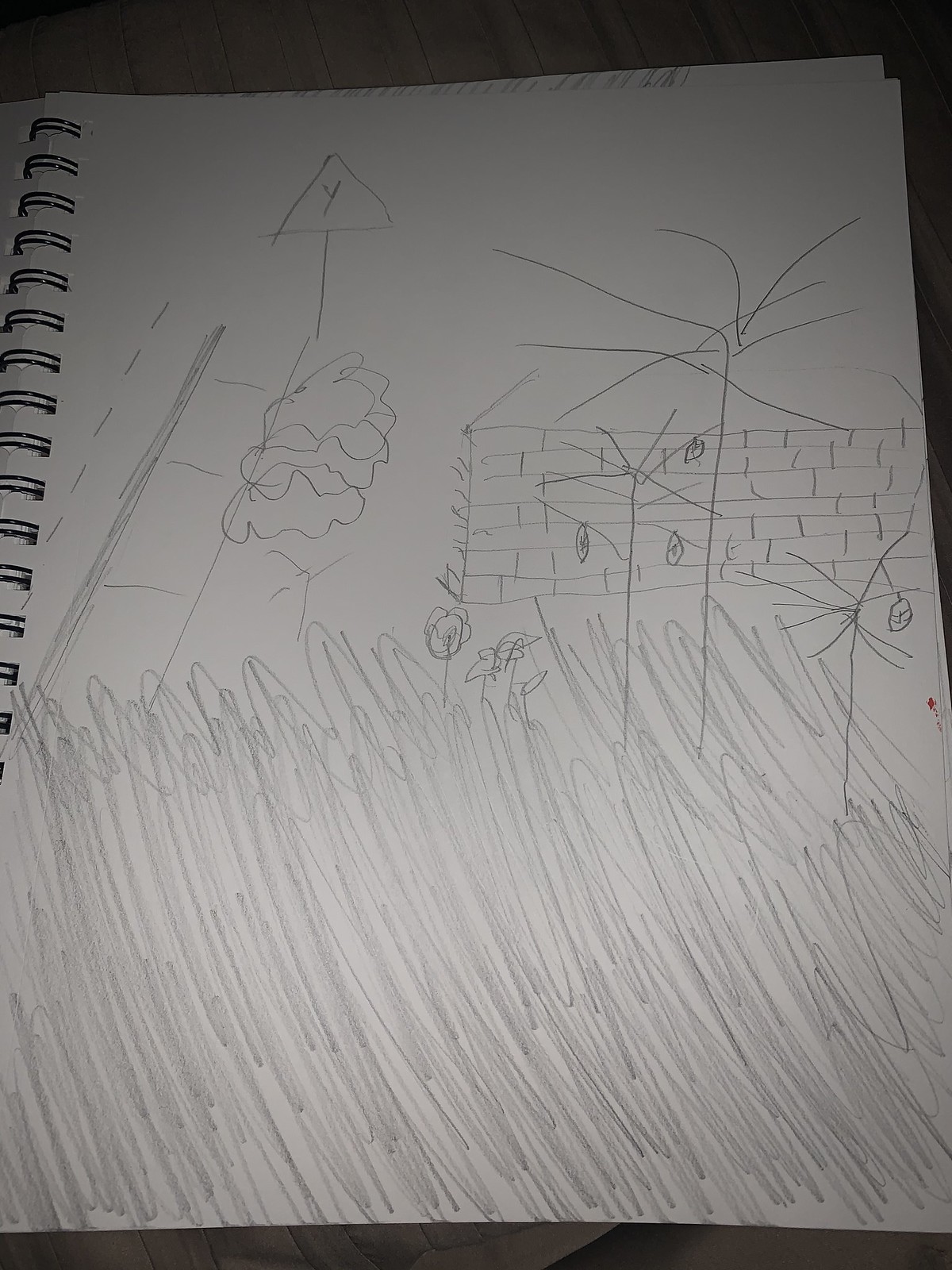A meticulously sketched black-and-white illustration adorns a spiral-bound notebook, the black spirals prominently visible on the left edge. The white pages starkly contrast against a seemingly dark background, possibly a table. The lower section of the drawing bursts with a flurry of penciled squiggles stretching from the right edge to the left and culminating in the center. Above these chaotic lines, various structured elements emerge: a solid line complemented by a broken one to its left, paired alongside several vertical lines intersected by horizontal dashes.

In the middle of these abstractions, a small flag is depicted, characterized by a straight pole, a triangular banner adorned with a central "Y," and underscored by whimsical cloud-like formations. Toward the right side of the page, the artist attempts a rudimentary house. This structure is outlined with what resemble brick patterns and crowned with a roof, detailed with fine lines radiating outward. The house is etched with lines crisscrossing its façade. Amid the frenzy of squiggles below, delicate flower-like shapes appear, their petals intricately sprouting from thin stems, adding a touch of organic charm to the otherwise surreal composition.